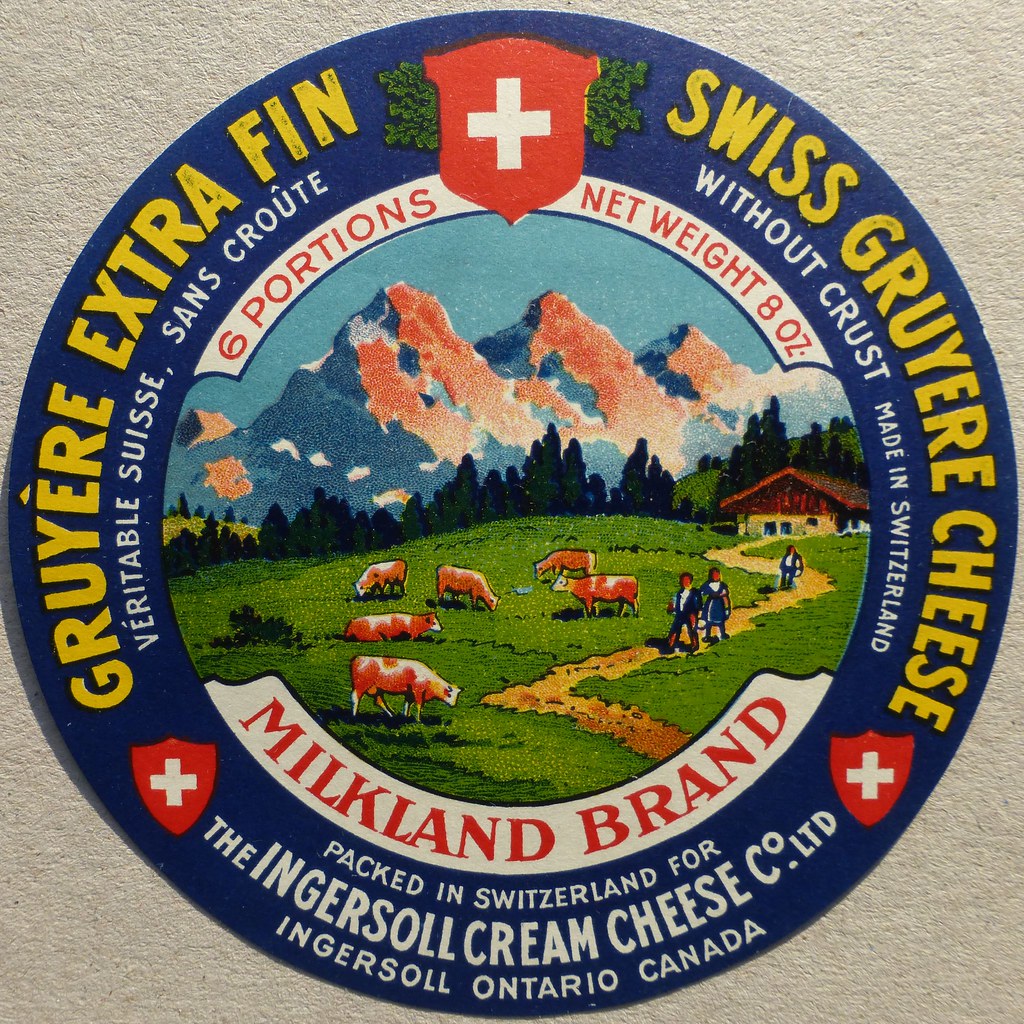This round sticker, predominantly blue, is for Milkland brand Swiss Guerrier cheese, which is without crust and made in Switzerland. The sticker features a prominent circular blue border adorned with red shields displaying white crosses. At its center, a picturesque farm scene is depicted, showcasing cows grazing in a green grassy field, farmers walking along trails, a barn, several trees, and snowy mountains in the background under a clear sky. The sticker indicates that the package contains 6 portions of cheese, weighing 8 ounces in total. It is packed in Switzerland for the Ingersoll Cream Cheese Co. Ltd., located in Ingersoll, Ontario, Canada. Additional text on the sticker, likely in a foreign language, specifies the type of cheese.